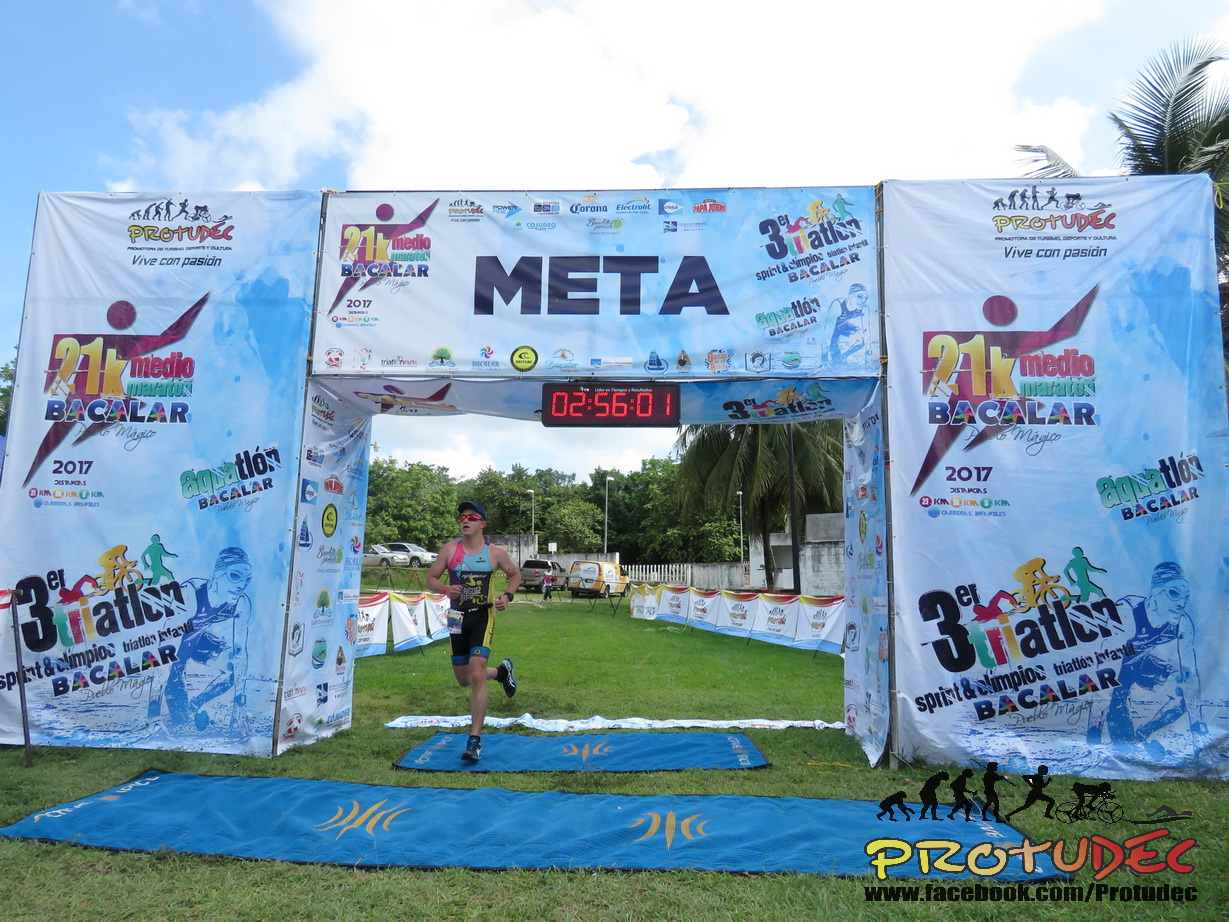In this image, a person is captured running through a finish line of what appears to be a marathon event. The finish line is marked by a large, light blue scaffolding archway covered with a tarpaulin that is adorned with colorful graphics and Spanish text. Prominently, the word "META" is displayed at the top of the arch in bold black letters, indicating the finishing point. The arch also features a digital clock showing a time of 2 hours, 56 minutes, and 1 second in red numbers. The event appears to be the "21K Marathon Bacalar," as observed on the tarpaulin.

The runner, dressed in a sporty tank top and running shorts that are primarily black and blue with some decals, crosses the finish line on a blue mat with a white stripe indicating the end. The runner is also equipped with a paper number pinned to their side, sunglasses, and a baseball cap. Surrounding the pathway are green trees, parked cars, and white fences lining the barricaded area with banners. The day is bright and clear, with blue skies and white clouds overhead, contributing to the vivid outdoor setting. Additionally, the logo for "Protudec" is visible at the bottom right of the photograph.